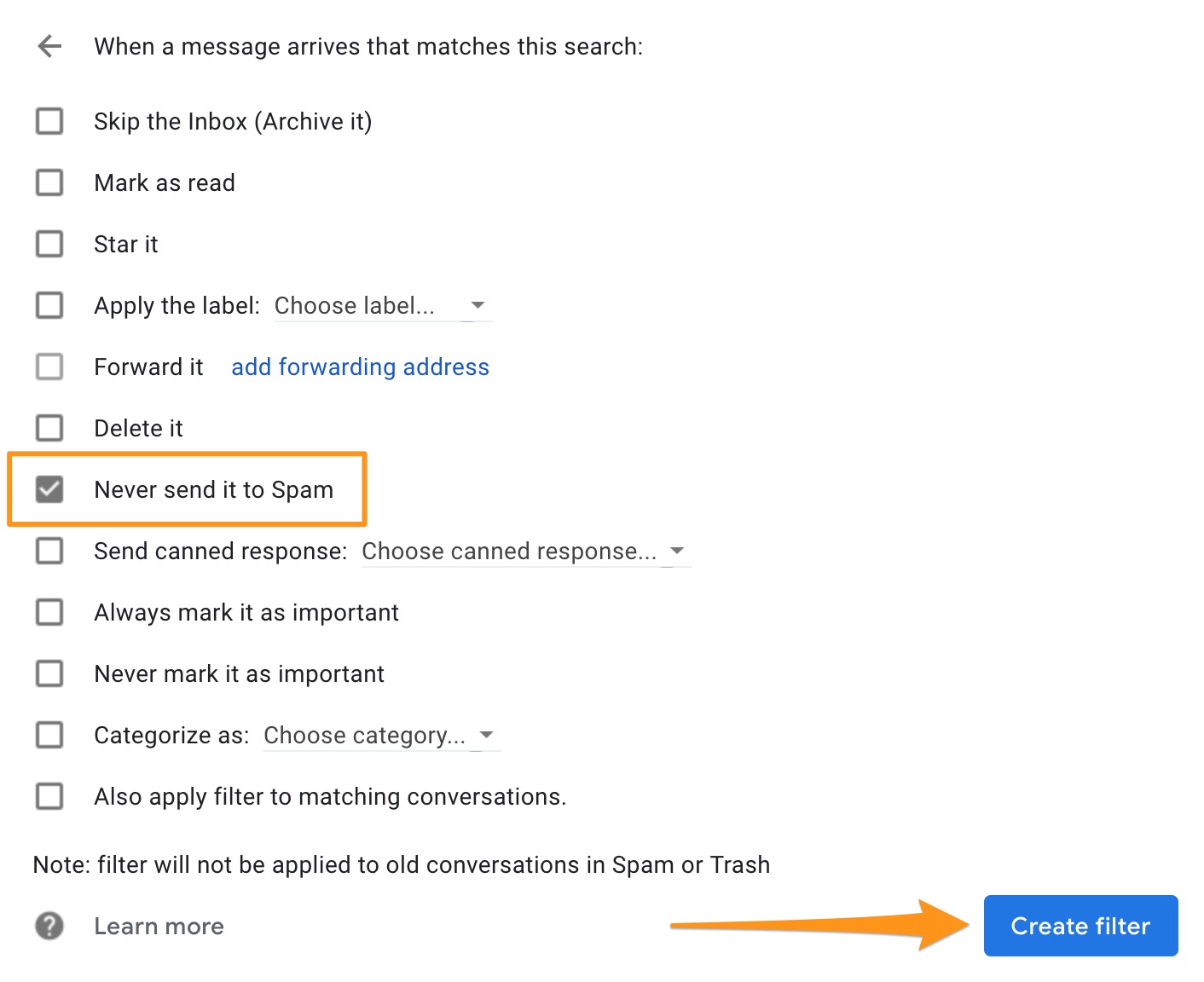The image features a screenshot of an email filtering settings menu with a white background. On the top left, there is a gray arrow pointing to the left, used for navigation. To the right of the arrow, the heading reads, "When a message arrives that matches this search:" with a capitalized "W" for "When."

Below the heading, there are twelve checkboxes, each accompanied by descriptive text. These options are as follows:

1. "Skip the Inbox (Archive it)"
2. "Mark as read"
3. "Star it"
4. "Apply the label: Choose label..." (includes a dropdown arrow for more options)
5. "Forward it" followed by blue text stating "Add forwarding address"
6. "Delete it"
7. "Never send it to Spam" (The checkbox is marked here, and this item is highlighted with an orange outline, indicating it is selected)
8. "Send canned response: Choose canned response..." (includes a dropdown arrow for more options)
9. "Always mark it as important"
10. "Never mark it as important"
11. "Categorize as: Choose category..." (includes a dropdown arrow for more options)
12. "Also apply filter to matching conversations. Note: Filter will not be applied to old conversations in Spam or Trash."

At the bottom left of the screen, there is a gray circle with a white question mark accompanied by the text "Learn more," with "Learn" capitalized. On the bottom right, an orange arrow points to a blue box containing the white text "Create filter," with "Create" capitalized.